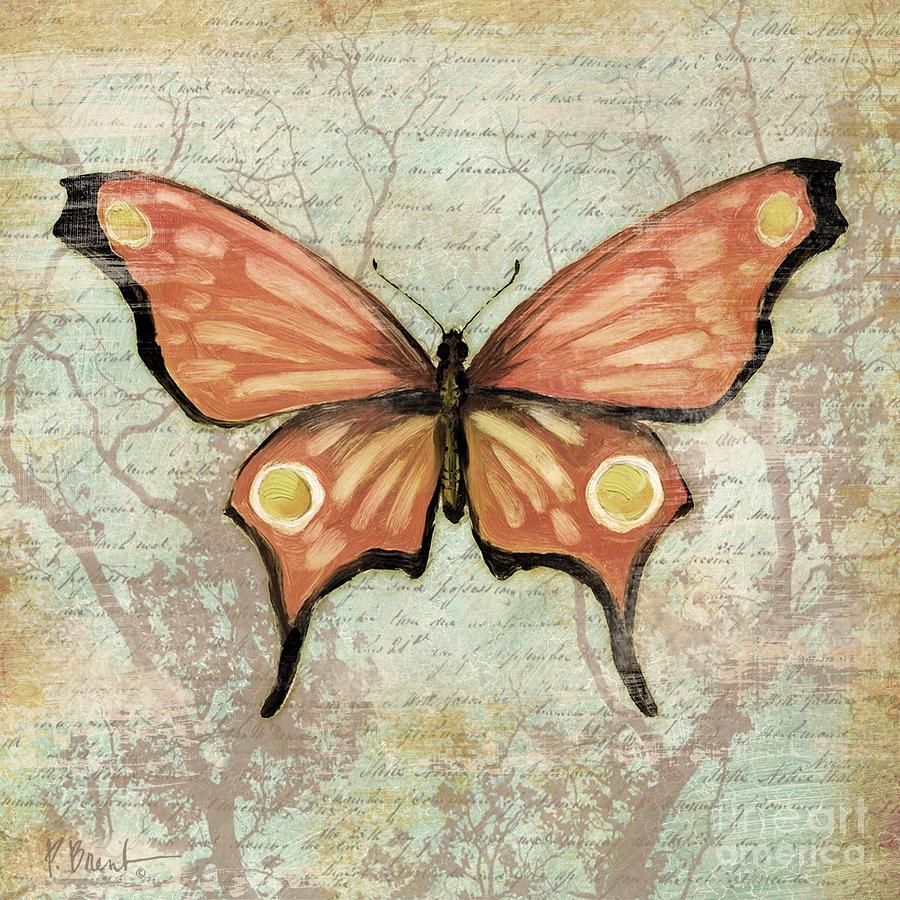This image features a detailed, colorful butterfly prominently centered on parchment-like paper. The butterfly, with a small black body and two visible black antennae, showcases vibrant orange wings accented with yellow dots near the corners and outlined with black. The intricate wings are made with broad strokes, giving it an artistic flair. Behind the butterfly, the parchment paper has faint traces of trees and cursive writing, reminiscent of historical documents like the Declaration of Independence, with hues of peach, green, and brown blending seamlessly into the background. The cursive text is illegible and covers the page delicately, adding an antique aesthetic. In the lower left corner, the artist's signature, "P. Brent," along with a copyright symbol, is visible. The bottom right corner includes what appears to be a dedication or phrase, with the words "heart America" discernible.